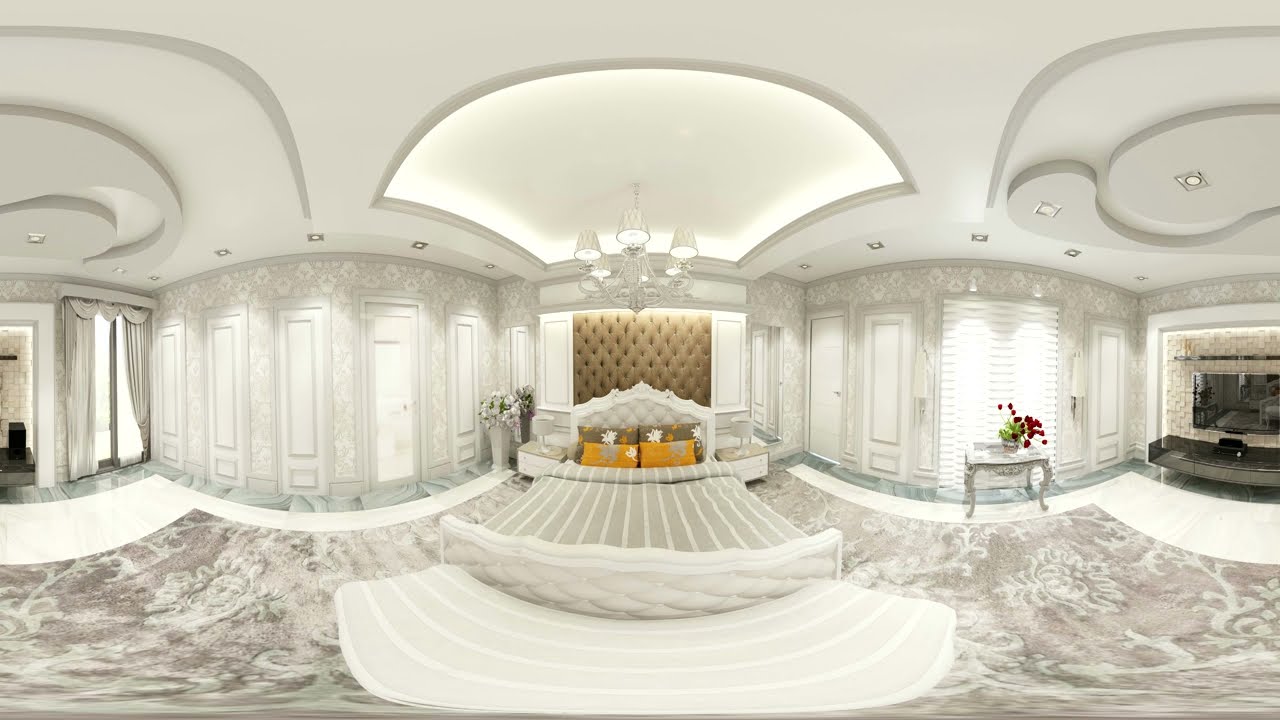The image captures the inside of an opulent and meticulously designed bedroom, predominantly adorned in shades of white and gray, epitomizing elegance and affluence. At the center of the room is a long bed with a headboard that features ornate woodwork and a fabric centerpiece with tacking. The bedspread is white with vertical light tan or grayish tan stripes, complemented by pillows in varying hues of orange, gold, and darker brown.

The room is impeccably well-lit, featuring a chandelier directly above the bed and several other lighting fixtures dispersed throughout, illuminating the luxurious details even during the night. To the right of the bed, there is a nightstand with a lamp and a small glass table showcasing a vase filled with vibrant red roses. A fireplace is nestled in the far-right corner, adding to the room's warmth and charm.

The floor is a blend of three distinct styles: a white rug with stripes front and center, bordered by a light copper-colored terrazzo flooring with a leafy white design, and white tiles leading to green tiles along the walls. The wallpaper is a very light gray adorned with a bone-white floral pattern that harmonizes with the room's classical paneling. A large window with a curtain drawn is positioned to the left, alongside what appears to be a sliding glass door, hinting at an adjacent bathroom.

This bedroom, likely belonging to a very wealthy individual, exudes luxury through its intricate details, from the floral designs on the floor and walls to the elegant furnishing and lighting, making it a paragon of sophisticated home design.